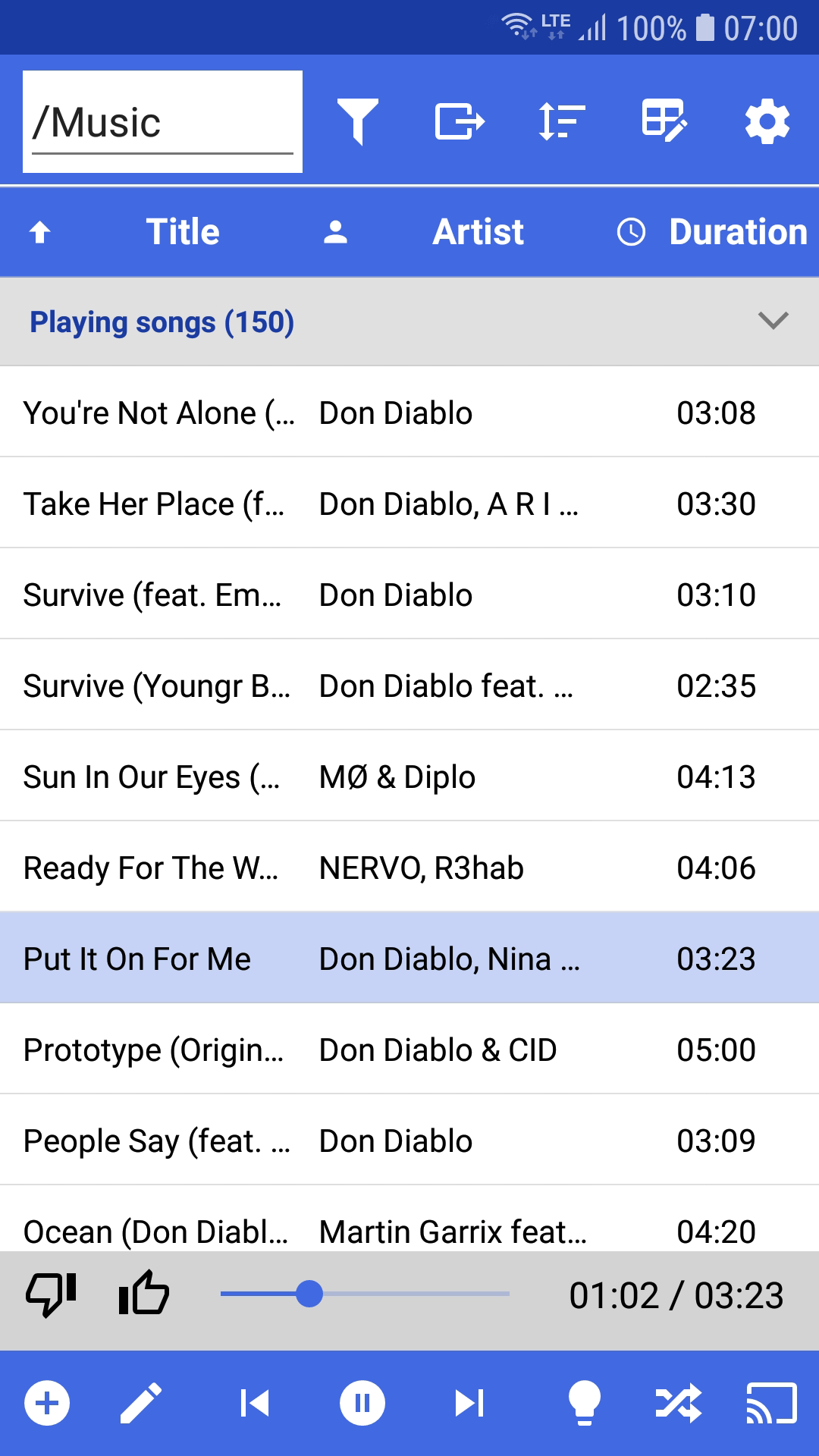The screenshot captures the interface of a music player app on a smartphone. The display is framed by a dark blue bar at the top, showing the status indicators: Wi-Fi strength, LTE connectivity, signal strength, a full battery icon labeled 100%, and the time reading 7 o'clock. Below this, a lighter blue stripe stretches across the screen. On the left of this stripe sits a white box with the text "/music”. To its right are several icons: one resembling a golf tee (function unknown), a forward arrow, a vertical arrow with arrows at both ends and three horizontal lines next to it, an icon resembling a window with a pencil, and a settings gear icon.

Another blue stripe runs horizontally, displaying an up arrow, a person icon, the title "Artist," and the label "Duration." Below this, a gray stripe reads "Playing songs 150," accompanied by a dropdown menu. The following list showcases song titles and artists:

1. "You Are Not Alone" - Don Diablo
2. "Take Her Place" - Don Diablo
3. "Survive" - Don Diablo
4. "Survive" - Don Diablo
5. "Sun In Our Eyes" - Emo and Diplo
6. "Ready For The Something" - Nervo and Rehab
7. "Put It On For Me" - Don Diablo
8. "Prototype" - Don Diablo
9. "People Say" - Don Diablo
10. "Ocean" - Martin Garrix

At the bottom of the screen, several controls are visible: thumbs down, thumbs up, a volume or scrubbing button, a plus sign, a pencil icon, and navigation buttons (back, pause, forward). Additional icons include a light bulb, a shuffle button, and a screencast option.